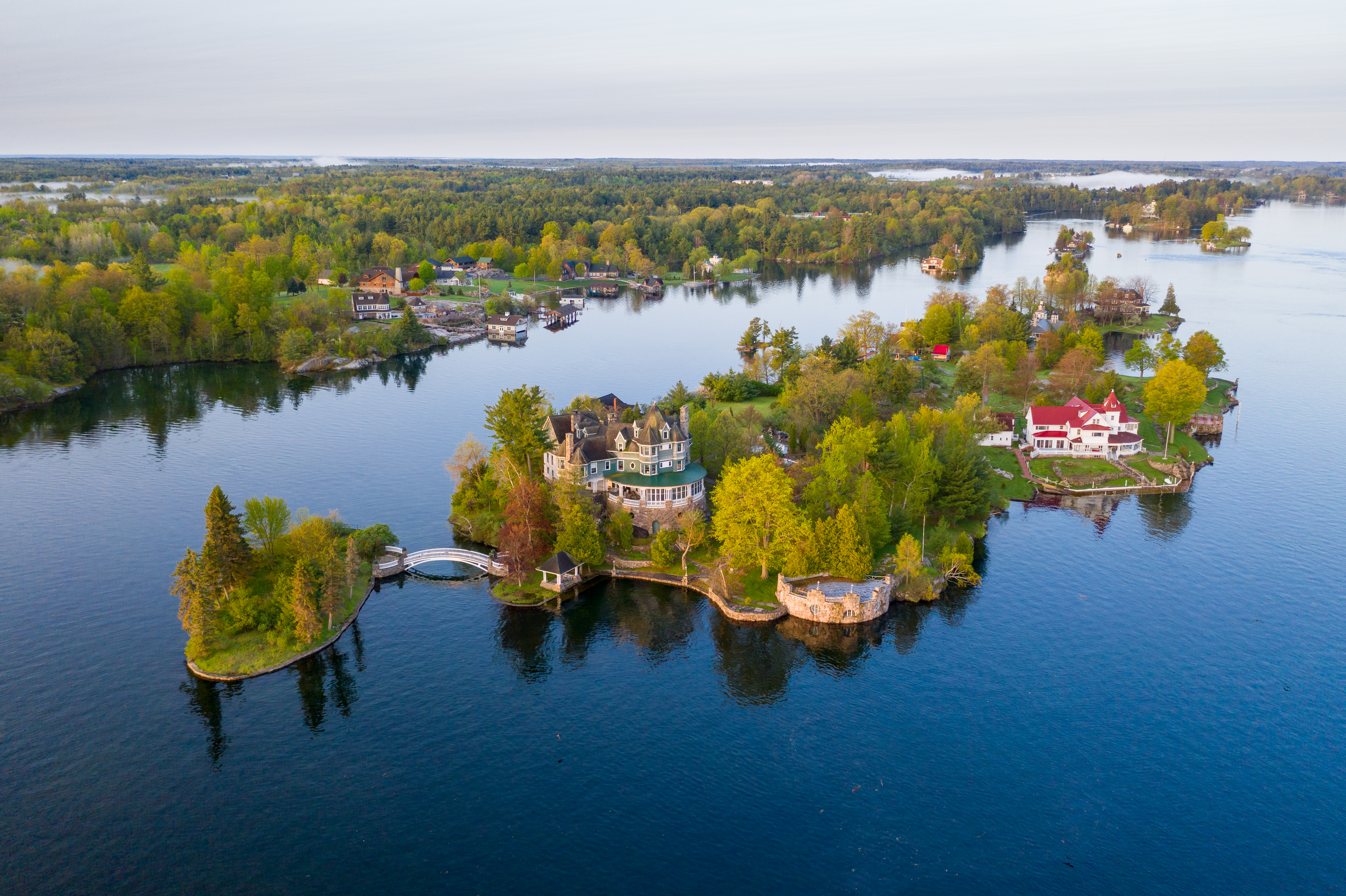This detailed aerial color photograph, taken in landscape orientation from a drone, captures a picturesque scene of a small chain of islands surrounded by a serene lake with varying shades of blue water. The main island, situated at an angle from the bottom left to the top right of the image, features three prominent structures nested amid lush, tall green trees. 

Dominating the foreground is a grand, castle-like mansion with a distinctive round shape, blue and brown turrets, and numerous windows, exuding a fairy-tale charm. Adjacent to this is a smaller, yet equally notable white house with a striking red tile roof near the middle right of the image. The island is also home to a quaint gazebo, adding to its idyllic nature. 

A graceful white arch-shaped bridge connects this larger island to a smaller, densely forested island on the left, enhancing the sense of a secluded haven. Beyond the islands, on the opposite bank of the river, is a verdant expanse of land covered in green trees, with a horizon line enclosing some ocean vistas, providing a peaceful backdrop to this captivating landscape. In the distance, on the top left of the image, other buildings and a small marina with several docked boats can be seen, adding a touch of civilization to the otherwise natural and serene environment.